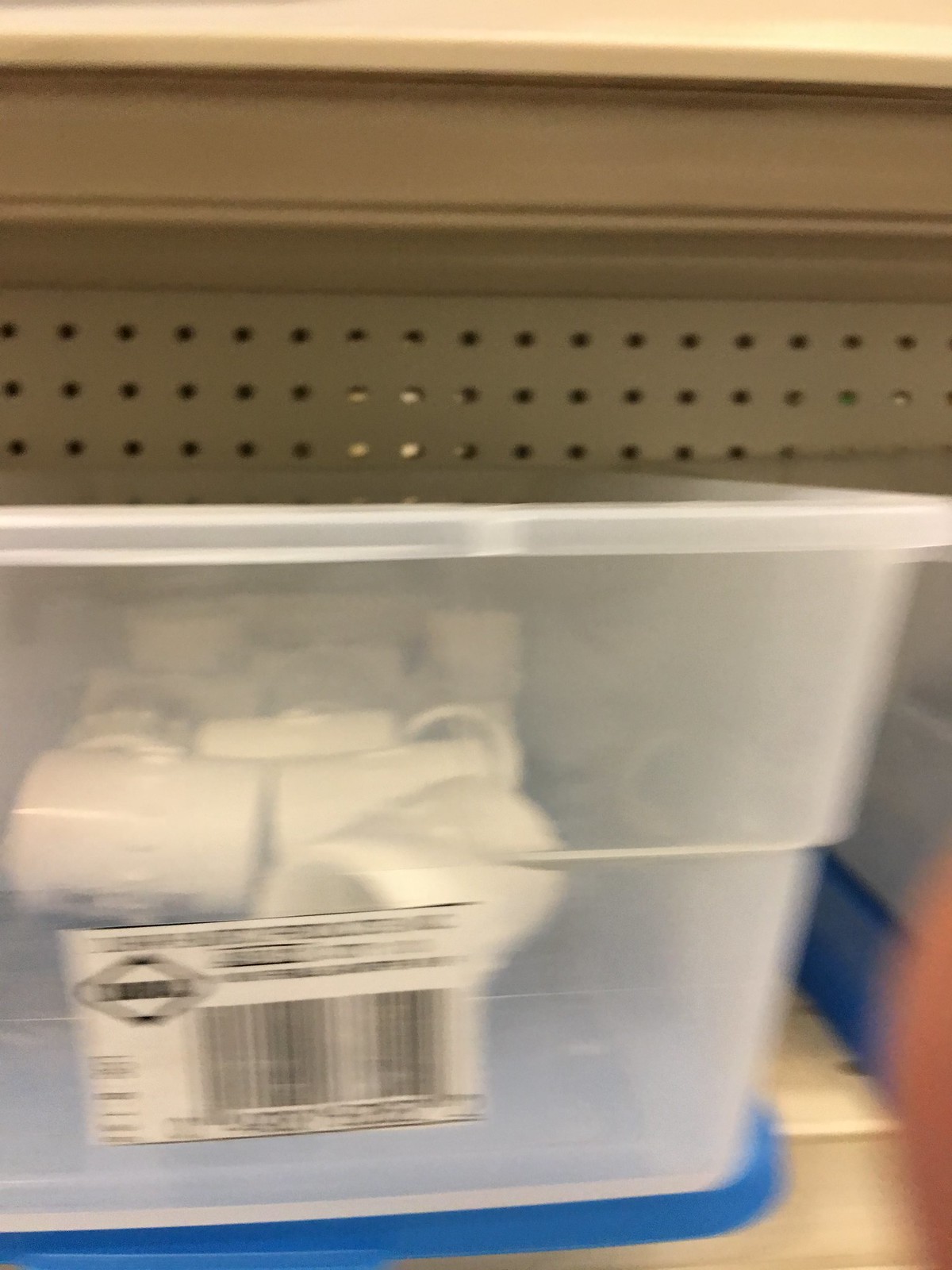The image displays a close-up view of a beige store shelf, characterized by a pattern of small circular perforations. The shelf has a gradient appearance, transitioning from light beige to a slightly darker beige and back to light beige again. Positioned on this shelf is a clear, rectangular storage bin. The handle of the bin, which is blue, appears to be situated underneath it. Attached to the bin is a white rectangle label featuring a black barcode. Although the specific text on the label is indiscernible due to the zoomed-in view, the barcode is clearly visible. Inside the clear bin, several white coffee mugs with matching white handles are stored. While the exact number of mugs is difficult to determine, at least four are clearly visible in the image.